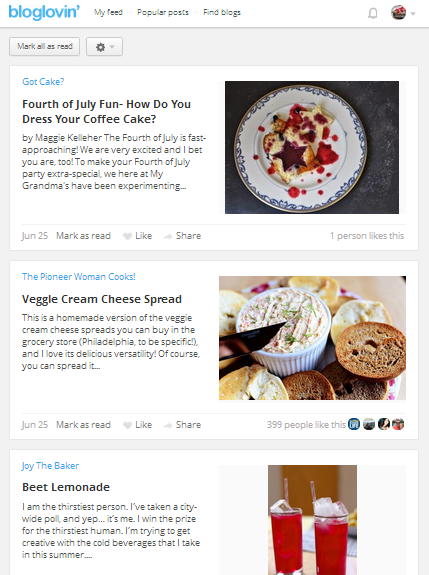This image showcases several articles from a food blog titled "Blog Loving," highlighted in blue at the top. The first article, written by Maggie Keller, is titled "God Cake, 4th of July Fun - How Do You Dress Your Coffee Cake?" It features a jelly-topped cake and discusses preparing for the upcoming 4th of July celebration, highlighting a family recipe. The second article, "The Poina Woman Cooks," presents a Veggie Cream Cheese Spread, a homemade version of the popular grocery store item, known for its delicious versatility. The final article focuses on a refreshing drink called "Beach Lemonade." The image captures the enticing variety of culinary delights and festive preparations featured on the blog.